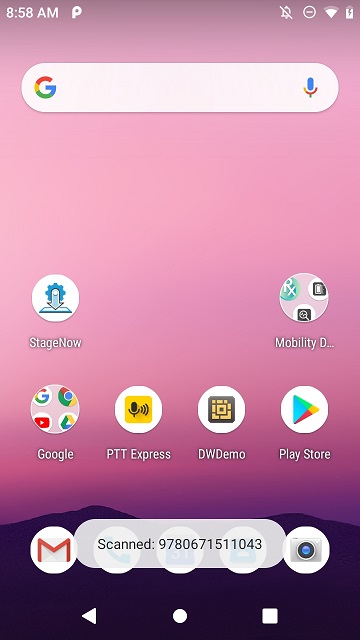This image displays a digital screen, potentially a tablet or a cell phone, showcasing various interface elements. The top left corner of the screen indicates the time as 8:58 a.m., while the top right corner includes a bell icon with a diagonal line through it, suggesting notifications are silenced. Adjacent to this is a "Do Not Disturb" symbol next to active Wi-Fi and charging battery indicators.

Dominating the top area of the screen is a Google search bar accented with the company's signature colors: red, yellow, green, and blue. The search bar also features a multicolored microphone icon on the right for voice search functionality. Beneath the search bar, app icons are arranged in a grid. The first row has an app labeled "Stage Now" on the left, with two empty spaces in the center, and an app named "Mobility D" on the right. 

On the second row, there is a Google app, followed by "PTT Express," "DWDDema," and the Play Store app. The third row includes a Gmail icon on the left and a Camera icon on the right, separated by a search bar displaying the text "scanned: 97806715111043." Below these icons are navigation buttons for the device: a left-pointing arrow, a circle, and a square, used for back, home, and multitasking functions, respectively.